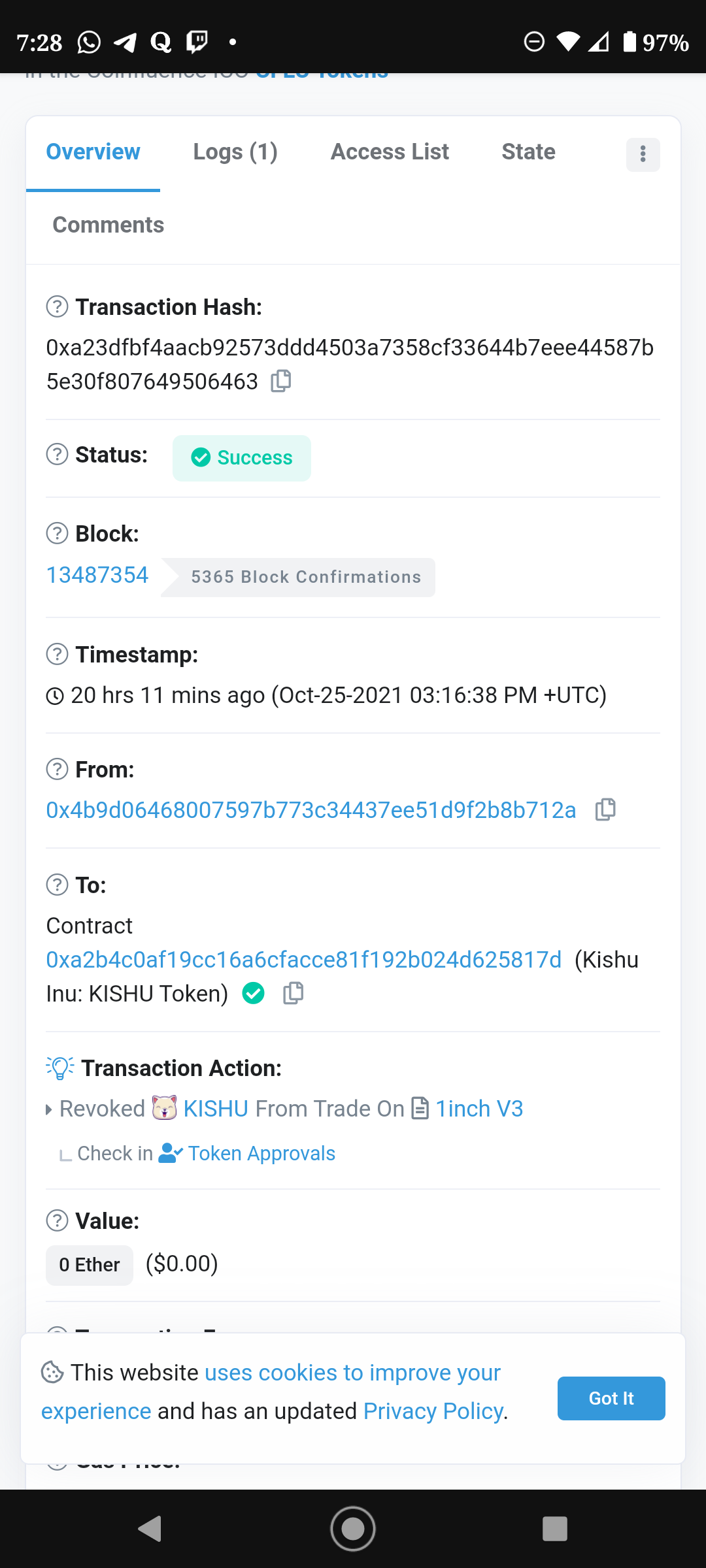This detailed screenshot from a mobile device captures a complex interface predominantly consisting of text, indicating some technical or financial data. The top of the screen displays the time (7:28), alongside various application icons such as Twitch, FaceApp, and Quora, as well as the status indicators for Wi-Fi, cellular signal, and battery level (97%).

The main section of the screenshot highlights a text-heavy dialog box with four selectable tabs at the top: "Overview," "Logs," "Access List," and "State," with "Overview" currently active. Below this, there are user comments, followed by a transaction hash composed of numerous alphanumeric characters, denoting a specific transaction identifier. The status of the transaction is marked as "Success."

Within the details, the transaction block number is identified as 13487354. Additionally, it includes a timestamp indicating it was recorded 20 hours and 11 minutes ago on October 25, 2021. The transaction value is specified as $0. However, numerous other data points are listed, which appear cryptic without additional context.

This screenshot is likely from a blockchain or cryptocurrency application, given the presence of transaction hashes, block numbers, and status indicators.